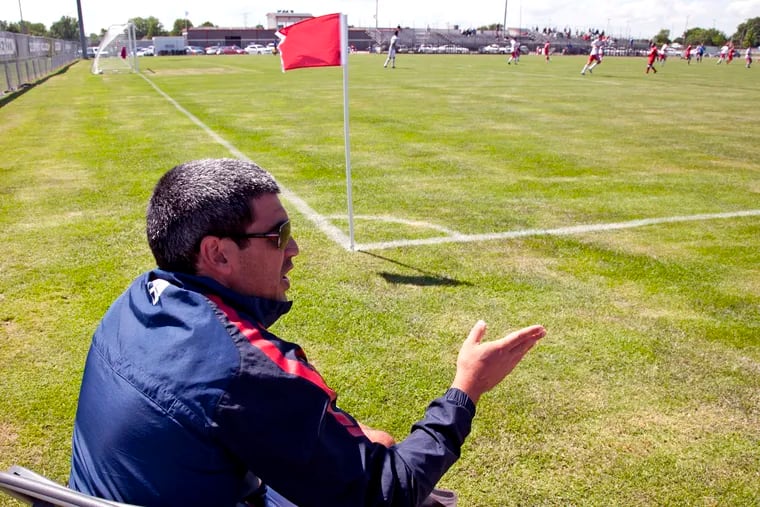In this daytime image, we see a man with short black hair, sunglasses, and a mustache sitting in a folding lawn chair at the corner of a fenced soccer field. He is dressed in a dark blue windbreaker adorned with a red stripe down the right sleeve. With his right hand extended as if making a point, he seems to be engaged in conversation with someone. The bright green field, enclosed by a six-foot chain-link fence, features white lines and arced sections in each corner, marked by white posts with red flags. Nearby, eight players in white shirts and red shorts are engaged in a soccer game. In the far background, a few buildings and parked cars are visible behind the fence, contributing to the overall scene. The sky appears white, casting a uniform light across the field.